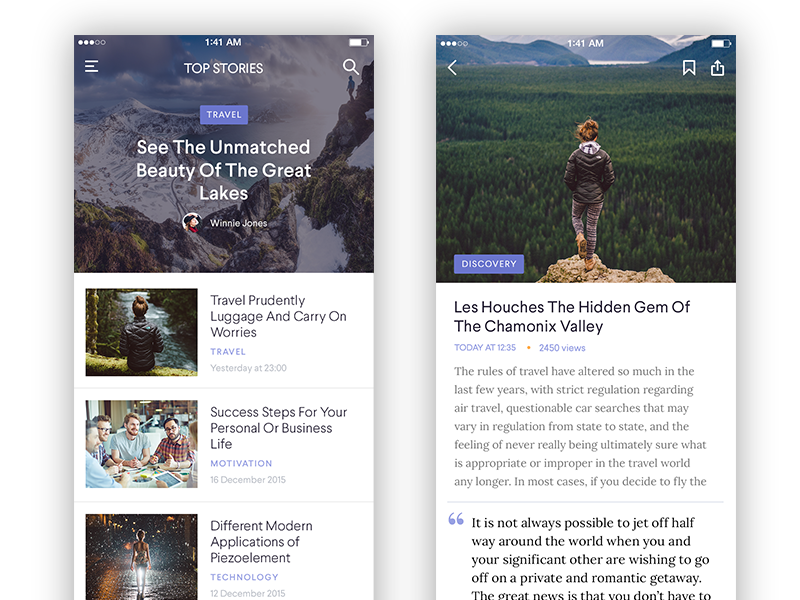Displayed in a magazine-style format, the two side-by-side images offer a visually compelling contrast. 

On the left side, the section titled "Top Stories" showcases an array of travel-related articles. Featured prominently is "See the Unmatched Beauty of the Great Lakes" by Winnie Jones, accompanied by various other pieces such as "Confidently Pack: Luggage and Carry-On Worries," "Success Steps for Your Personal or Business Life," and "Modern Applications of Piezo Elements." Each article is accompanied by stock photos, most depicting outdoor scenes.

On the right side, an evocative image captures a woman standing on a rocky outcrop, gazing over a vast forest expanse. The text reads, "Les Houches: The Hidden Gem of the Chamonix Valley," suggesting a focus on this picturesque location. The article likely delves into the challenges and changes in travel regulations over recent years, with a specific emphasis on air travel and car search protocols. The awe-inspiring natural scenery contrasts sharply with the detailed section titles and stock photos on the opposite side, creating a dynamic composition that marries the allure of travel with practical advice and fascinating topics.